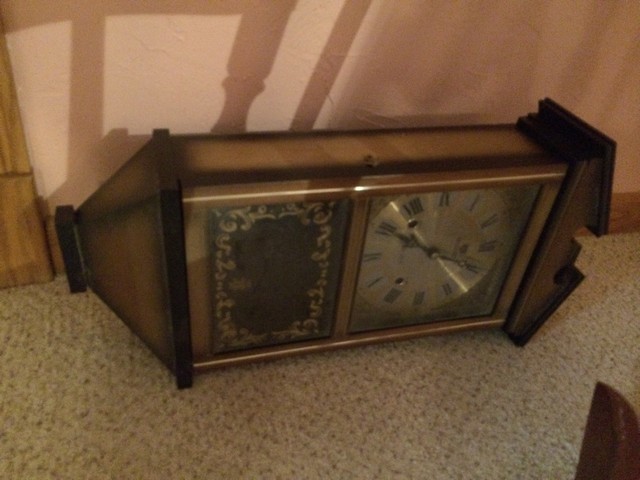This is a color photograph of an antique wooden cuckoo clock that is turned on its side, with the clock face facing to the right. The clock is made from wood that features a gradient from dark to light tones. The clock face is silver with black Roman numerals and black hands, encased in a round window with a square wooden frame and a detailed Victorian gold border surrounding a black area below it. The bottom half of the clock includes a clear glass door with ornate gold scroll patterns. The clock is resting on a textured, short beige carpet with black speckles. The background reveals a mildly pink wall with a light natural wood trim at the base, and to the left, wood trim climbing vertically, likely part of a door or furniture, casting shadows on the wall that suggest a nearby railing, possibly from a staircase.